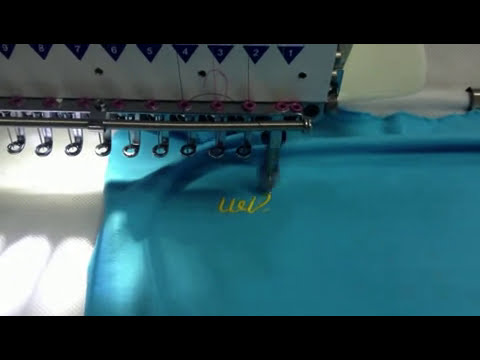The photograph depicts a detailed close-up of an embroidery machine, presumed to be a sophisticated model with at least 10 needle points. The machine’s metallic silver components are visible, particularly where the needles align and possibly descend to perform stitching. The machinery is partially draped in white fabric adorned with blue triangles, adding a decorative element. Positioned beneath the machine, a blue piece of fabric is being embroidered with yellow threads, likely forming initials or letters, as suggested by the visible characters. This blue fabric sits atop another layer of white fabric or perhaps a white table. 

Above the main fabric surface, the machine showcases several silver hooks or loops, guiding the thread through its intricate threading system. Additional details such as measurement indicators can be noted on the machine, emphasizing its precision and functionality. Sunlight streams into the image, slightly obfuscating some details but highlighting the machine and the fabric. The photograph lacks human presence, focusing solely on the embroidery process. The overall image quality is medium, captured within a frame roughly 5 inches wide by 4 inches tall.